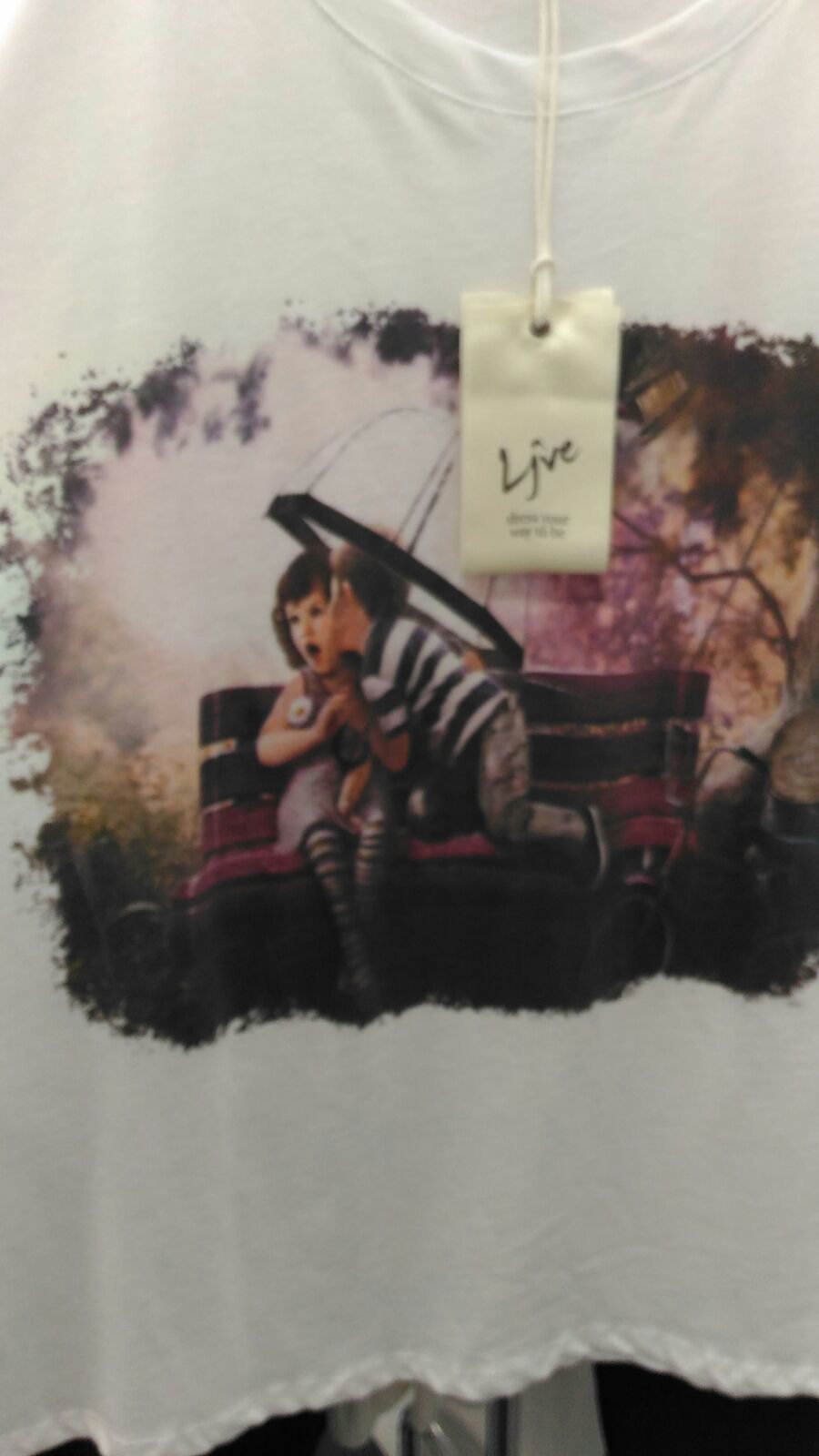The image is a detailed photograph of a white t-shirt for sale. The t-shirt prominently features an image printed in the center, depicting a tender scene of a young boy and girl on a deep burgundy park bench. The boy, who has short brown hair and is wearing a white and black striped shirt along with tan pants that fall just below the knees, is sweetly kissing the girl on her left cheek. The girl, with dark hair styled in pigtails, is seen in a lavender tank dress with black and white striped stockings. She holds an umbrella, hinting that it might be raining, and appears to be shocked by the kiss. The bench they sit on has a soft pink and lavender background. Additionally, hanging over the top of the image on the t-shirt is a light beige tag that reads "LIVE," although the smaller text beneath is not legible. This detailed scene captures a touching moment between the two children.